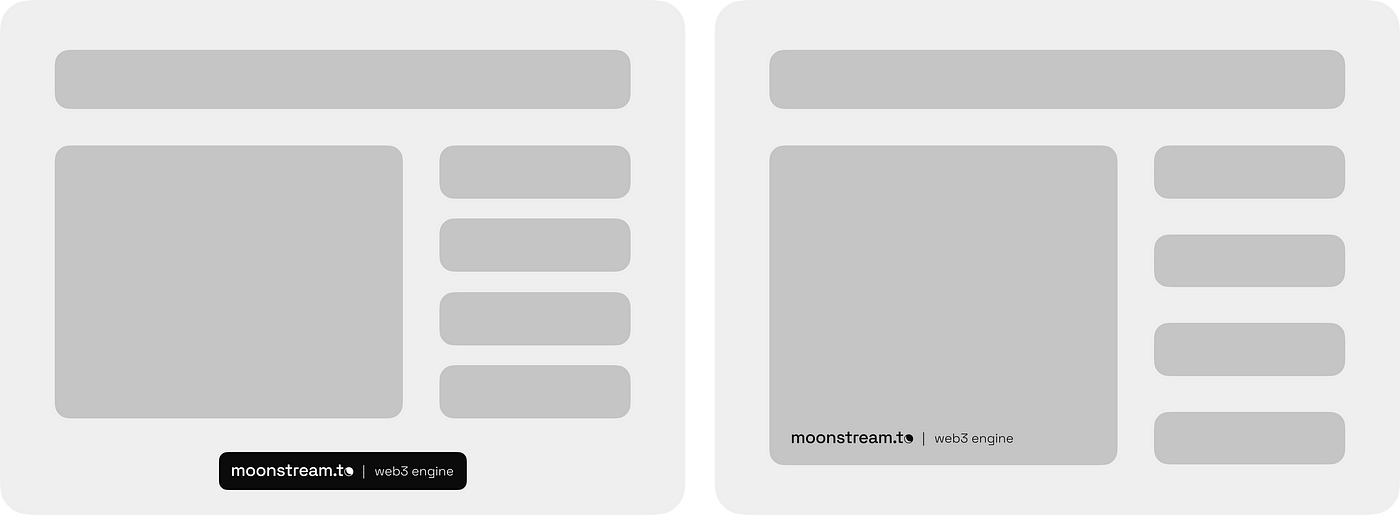This set features two minimalist-styled images with a light gray background, designed to mimic a user interface. Each square image, both with rounded corners, has a composition of dark gray horizontal lines: a longer line at the top and four shorter lines aligned to the right, simulating text. On the left side of each image, a gray square suggests a placeholder for a photo. Notably, the image on the left includes an additional black rectangle at the bottom that reads "Moonstream.to Web 3 Engine". The right image exhibits this same text within the gray square at the left side. The images are purely abstract with no photographic elements, showcasing no presence of people, animals, plants, buildings, vehicles, or any other tangible objects.